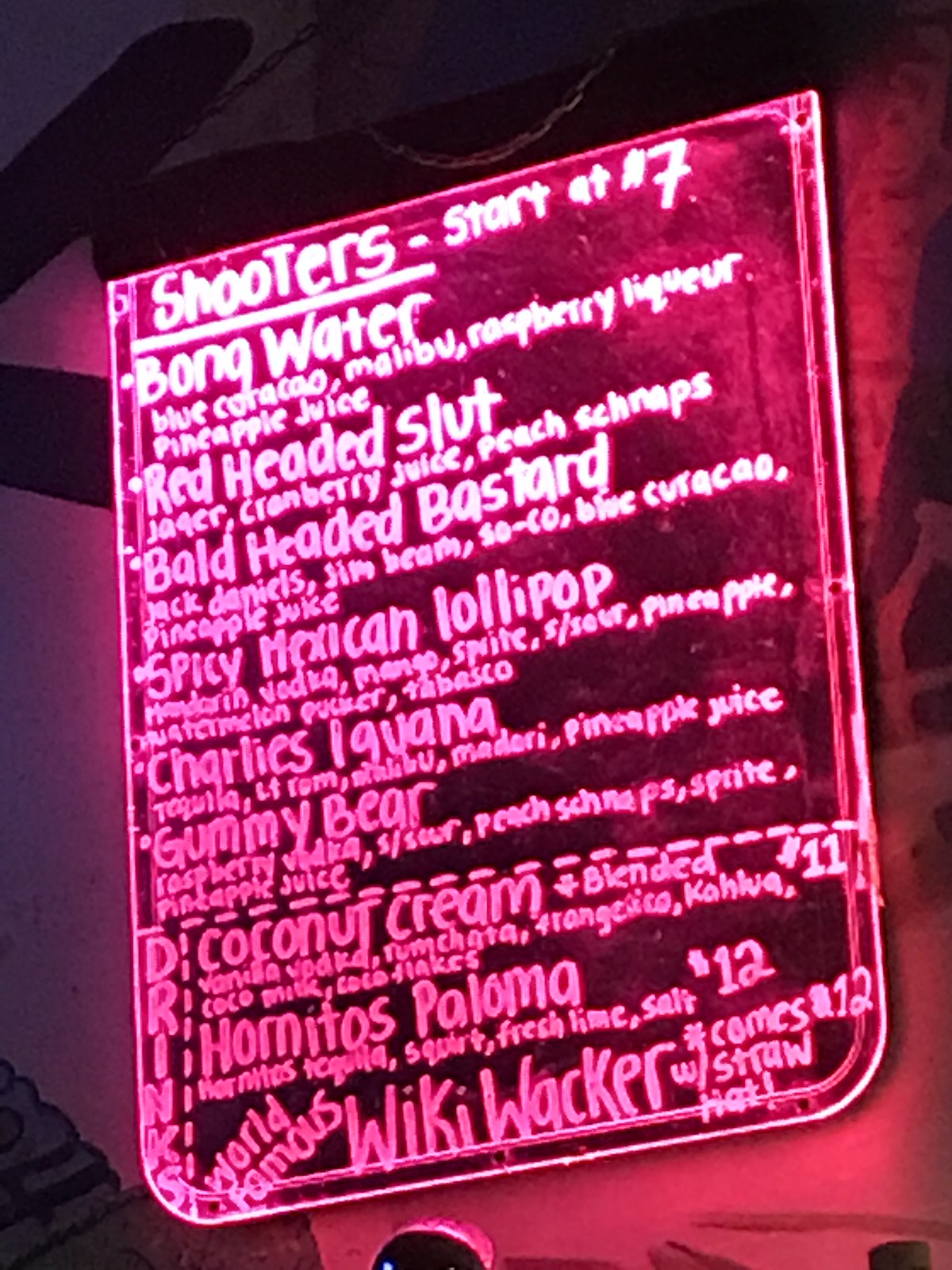This photo captures a vividly-lit, rectangular neon sign with a pink luminescence, advertising drink specials at what appears to be a bar. The sign, observed at a slight angle, is predominantly black but illuminated by a vibrant pink light. The text on the sign, seemingly white but glowing pink due to the lighting, lists various drinks with humorously inappropriate names.

At the top, the word "Shooters" is prominently displayed and underlined, followed by the notation "start at $7." Below this heading, a variety of shooters are listed in large fonts, with ingredient details in smaller fonts. The first shooter is named "Bong Water," followed by "Redheaded Slut," each with a description of their ingredients. Continuing down the list are creatively named concoctions such as "Bald-Headed Bastard," "Spicy Mexican Lollipop," "Charlie's Iguana," and "Gummy Bear."

At the very bottom edge of the sign, the word "Drink" is noticeable, introducing another section of drinks. These include "Coconut Cream" priced at $11 and "Cornitos Paloma" priced at $12. The final item on the menu is the "World-Famous Wiki Whacker," which is noted to come with straw hats and is priced at $12.

This engaging and whimsical sign provides a snapshot of the bar's spirited and lively atmosphere, offering an array of distinct and amusingly-named shooters and cocktails.